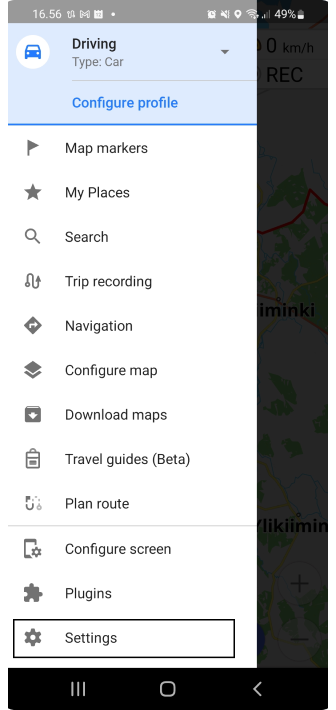The image is a screenshot from a mobile application on a smartphone. The bottom of the screen features a black navigation bar with three white vertical lines representing the menu option, a square icon for the home button, and a left-pointing arrow for the back button. At the top of the screen, a gray status bar displays the time as "16:56," along with several status icons, including the Gmail logo, an alarm clock, a muted sound indicator, a GPS icon, data and Wi-Fi connectivity icons, and a battery icon showing 49% remaining battery life.

Below the status bar, there is a blue pop-up window labeled "Driving," featuring options such as "Type Car" and "Configure Profile." A white circle with a blue car icon is prominently displayed within this window. Below the pop-up, a list of menu options is visible: "Map Markers," "My Place," "Search," "Trip Recording," "Navigation," "Configure Map," "Download Maps," "Travel Guides (Beta)," "Plan Route," and "Configure Screen." Additionally, there are options for "Plug-ins" and "Settings," with "Settings" being highlighted, indicating that it is currently selected.